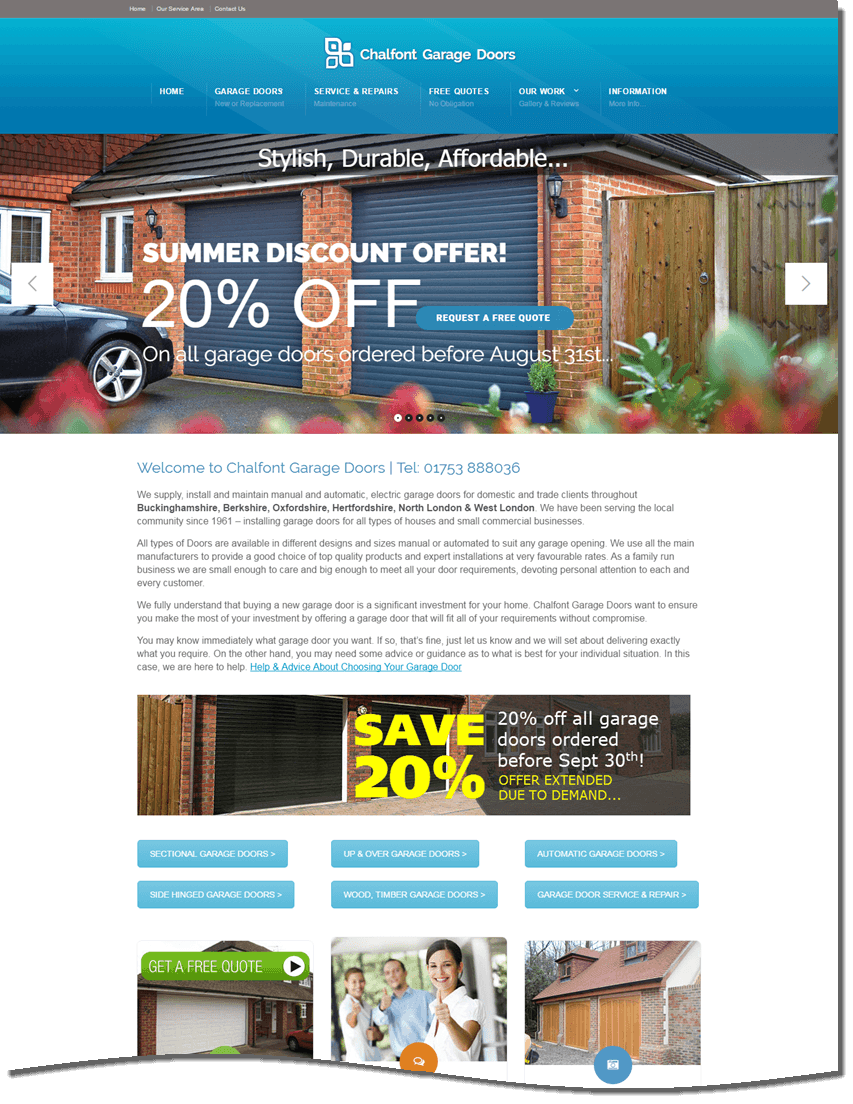This promotional image for Chalfant Garage Doors showcases a sleek and user-friendly website interface. The design features a wavy, decorative border. At the top, there is a prominent blue banner displaying the Chalfant Garage Doors logo, accompanied by navigation buttons for Home, Garage Doors, Service & Repairs, Free Quotes, Our Work, and additional information.

In the primary banner section, a high-quality image of a garage with a car parked in front displays with white text detailing a summer discount offer: "Stylish, Durable, Affordable. Summer Discount Offer, 20% Off." It includes a call-to-action button labeled "Request a Free Quote" and reiterates the 20% discount on all garage doors ordered before August 31st.

The website welcomes visitors with a message: "Welcome to Chalfant Garage Doors." It provides their contact number, 01753-888-036, and highlights their services, which include the supply, installation, and maintenance of manual and automatic electric garage doors for both domestic and trade clients throughout Buckinghamshire, Berkshire, Oxfordshire, Hertfordshire, North London, and West London. The company boasts a long-standing history in the local community, having served since 1961.

A secondary banner below the main content emphasizes an extended offer: "Save 20%. 20% Off on all Garage Doors ordered before September 30th, author extended due to demand." Following this, users can explore various types of garage doors via clearly marked buttons, facilitating an easy and comprehensive browsing experience.